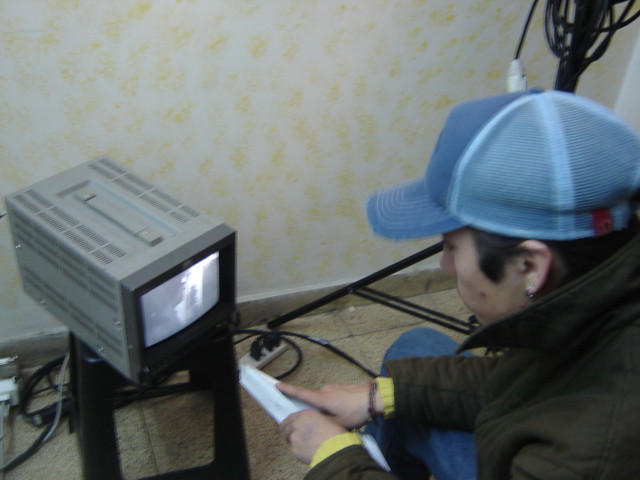In the photograph, we see a man seated on the right side, wearing a blue baseball cap and a dark down jacket, engrossed in examining a small, black-and-white monitor. The monitor, which resembles an old-fashioned TV screen, is placed on a footstool and displays an indistinct image that looks like a pair of legs, possibly someone dancing. The man is holding a notebook or a sheet of paper, likely related to his work, suggesting he might be a video technician. The setting appears to be an indoor space with a carpeted floor and a plaster wall in the background. Various wires can be seen, including several connected to a plug on the wall and a coiled wire hanging from a pole. The scene features a muted color palette of white, yellow, gray, blue, and black.